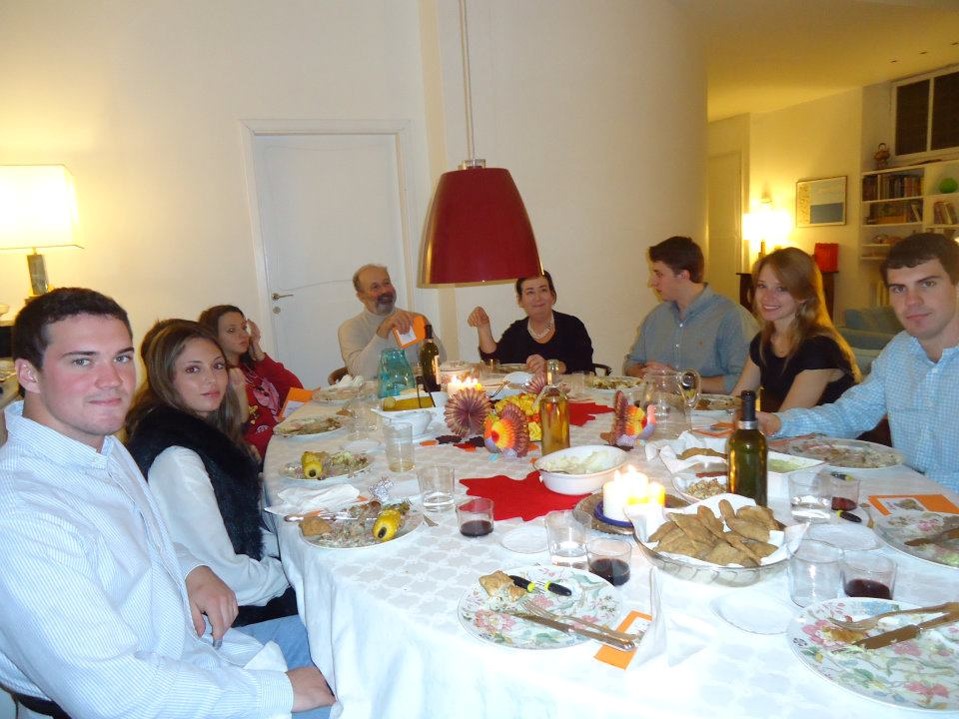A vivid full-color square photograph captures a joyful family meal taking place indoors under artificial lighting. The focal point is an oval table draped with a white tablecloth, set for what appears to have been a festive occasion, perhaps Thanksgiving given the themed center decorations. Nine people are seated around the table, which is arranged with floral print plates, some still holding partially eaten corn cobs. The room has white walls, and notable lights include two lamps on the sides and a prominent red-shaded pendant light hanging above the table, though it is not lit.

At the head of the table sits an older man in a beige turtleneck, beside an elderly woman with a pearl necklace and pixie-cut black hair, clad in a black shirt. The rest of the table is occupied by what seem to be their adult children and possibly their partners. On one side, a man in a white shirt sits next to a woman in a white shirt and black vest, followed by a dark-haired individual obscured from full view, and a woman in a red sweater. The other side features a younger man in a button-up shirt, a woman in a black shirt, and a dark-haired young man also in a button-up shirt. The patriarch is notably wearing a mask, which is not worn by any of the others. The table is adorned with three bottles of wine, contributing to the sense of a well-enjoyed meal among a happy family.